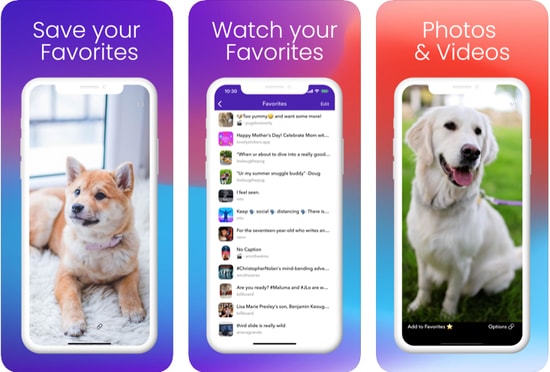The image montage features three side-by-side vertical images of cell phones, each outlined in white. The first two images share a gradient background that transitions from dark purple at the top, through a pinkish orange-red and sky blue, to purple at the bottom. 

In the leftmost image, a husky-mixed puppy lies on a white bed in front of a window, with the text "Watch Your Favorites" prominently displayed. The phone has a dark purple banner at the top, but the text and icons are too small to discern.

In the center image, similarly outlined and bannered, the gradient background remains consistent with the first, but it features a column of unreadable icons on the left against a white backdrop. A black sentence next to the icons describes them, though it is illegible.

The third image diverges with a solid color background: orange at the top and turquoise blue at the bottom. It also features a white-outlined phone, this time displaying a white dog resembling a Labrador retriever sitting in a grassy yard, looking off to the right. Small white text at the bottom remains too tiny to read.